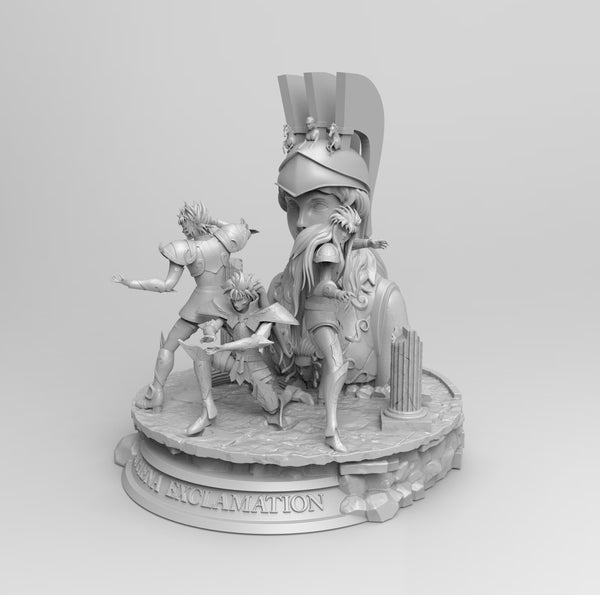The image depicts a detailed silver sculpture, likely reminiscent of ancient Roman or Greek artistry, featuring three warriors and a prominent helmeted bust set against a complex base. The base, round with a stone-trimmed edge, includes an engraved inscription, partially readable as "exclamation." The top of the base mimics a stone surface with broken pillars. At the center of the display is a bust of a figure wearing a traditional Roman helmet adorned with three distinctive plumes, with intricate details including a depiction of two horses and a central figure between the flares. Positioned in front of the bust are three distinct warriors in varying poses: one stands with arms raised, another is bent on one knee, and the third, appearing to be a female, is in a defensive stance. Each warrior is clad in ornate armor with exaggerated shoulder protectors, and their designs seem to draw inspiration from both historical and anime styles, featuring dramatic, spiky hairstyles.